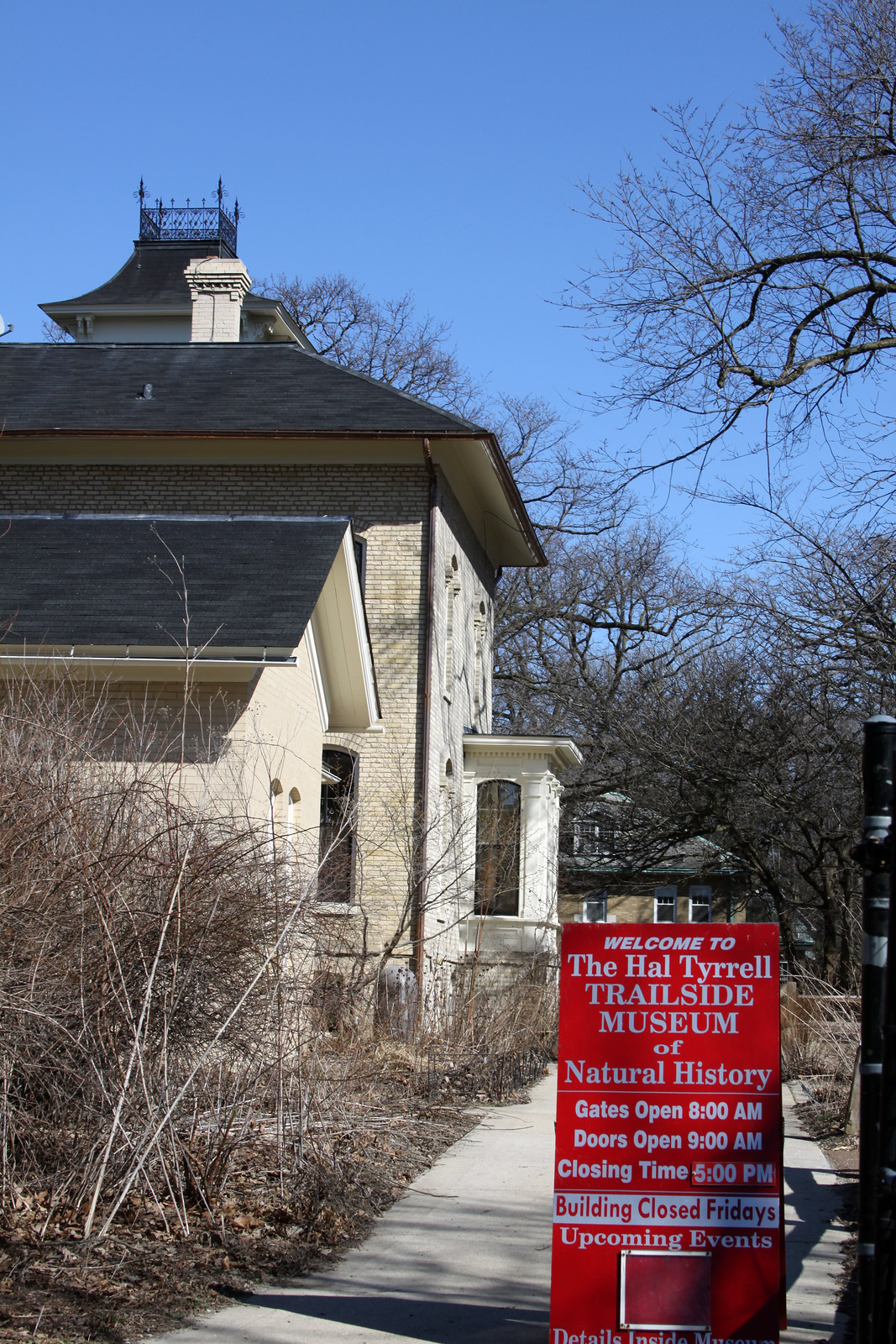In the image, the centerpiece is the Hal Tyrell Trailside Museum of Natural History, situated against a backdrop of a clear, cloudless blue sky. The museum itself is a multi-story structure made of white and light brown brick, capped with a black roof featuring a chimney. A sidewalk runs to the right of the building, while the left side of the structure is complemented by dense, leafless trees, suggesting a fall or winter season.

A prominent red sign with white text, located on the lower right corner near the sidewalk, welcomes visitors to the museum. The sign provides essential information: "Gates open 8 a.m., Doors open 9 a.m., Closing time 5 p.m., Building closed Fridays, Upcoming events." The notice about the building being closed on Fridays is highlighted with a white background and red text. Below, a smaller note reads, "Details inside."

Additional context reveals another building in the background that resembles a house, complete with windows and a roof. Overall, the clear sky, stark trees, and detailed signage create a vivid, informative scene inviting visitors to explore the museum.